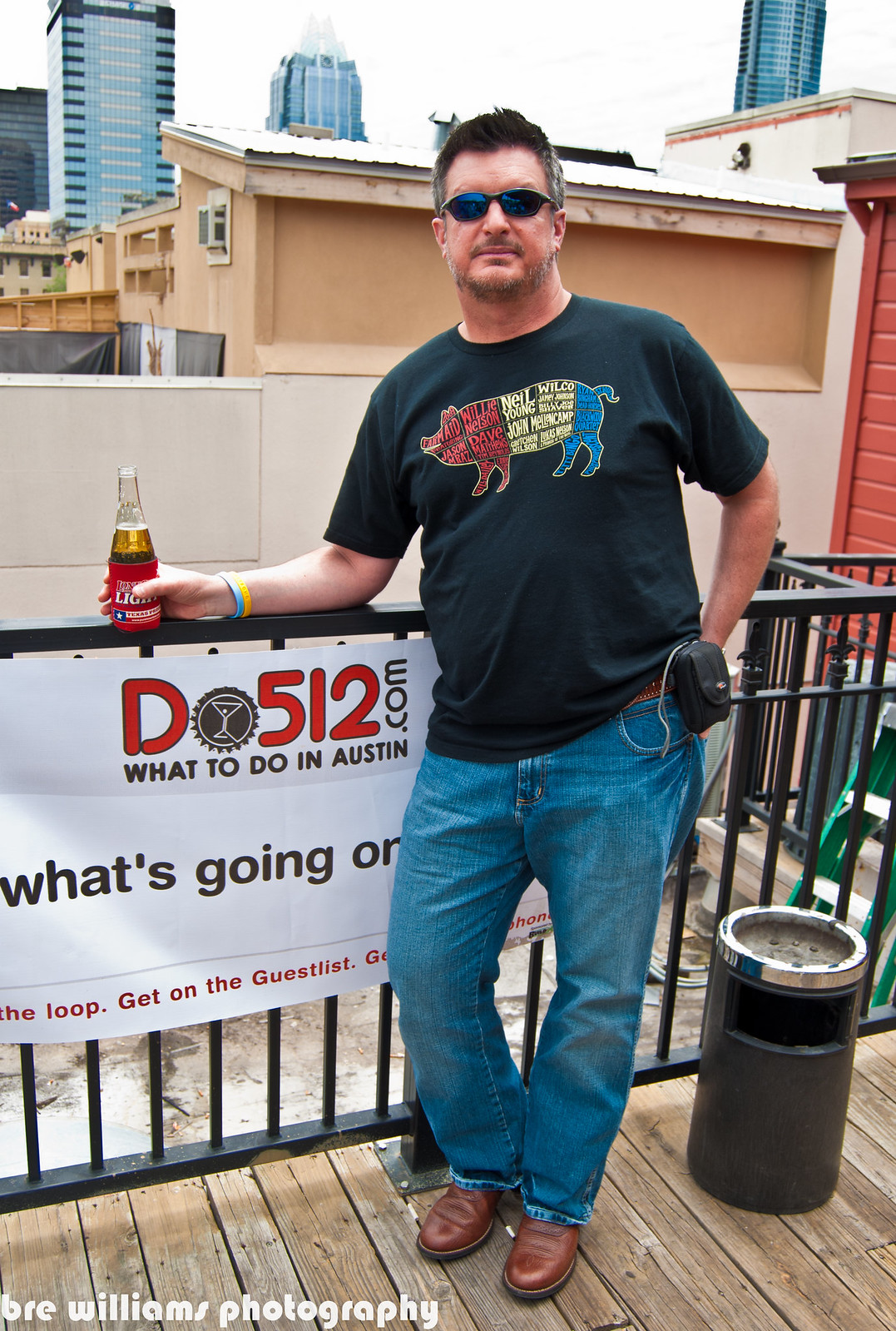This tall, vertically oriented outdoor photograph captures a man enjoying a relaxed moment, leaning against a black metal railing on a gray wooden deck. The man is positioned slightly to the right of the image, wearing reflective blue sunglasses, a black T-shirt depicting a pig colored with red, yellow, and blue text, blue jeans, and brown leather shoes. His right arm extends to rest on the railing, holding a beer bottle encased in a red holder. Two entry bracelets are visible on his wrists. Behind him, spanning the width of the gate, is a white banner that reads "DO512.com, What to do in Austin." To his right stands a black, cylindrical ashtray with a chrome top, for smokers. 

In the backdrop, the upper part of the image showcases a city skyline with several blue and black high-rise buildings. Below these are shorter, gray buildings. On the right edge of the frame, the red facade of another building peeks into view. At the bottom of the image, the credit "Bree Williams Photography" is subtly displayed, giving acknowledgment to the photographer. The entire scene exudes a casual, laid-back vibe, capturing a man indulging in a peaceful, easy-going moment in Austin.